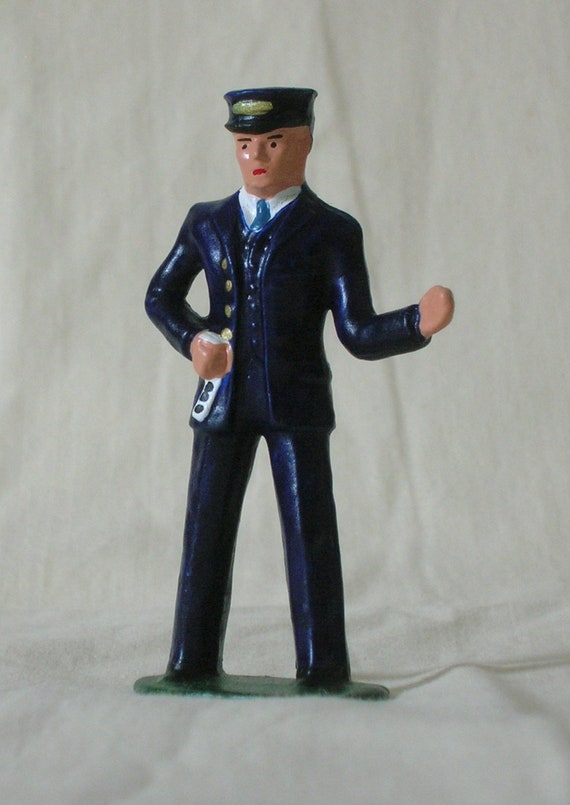This image portrays a small, historically styled ceramic figurine of a train conductor, situated against an off-white or white fabric backdrop. The figurine features a dark blue or very light black uniform, consisting of a suit jacket adorned with gold buttons, a vest, and matching pants. Completing the attire is a dark blue conductor's hat with a small gold emblem, a white button-up shirt, and a blue tie. The figurine's facial details are minimal, comprising light pink skin, a red line for the mouth, simple black dots for the eyes, and thin black lines for eyebrows. The conductor's right hand is extended as if to signal stop, while the left hand holds an indistinct object, possibly a bottle, near the waist. The legs of the figure are joined by a green platform that allows it to stand. Despite the lack of contextual information or scale indicators in the image, the weathered appearance of the figurine suggests it could be an antique piece of art.